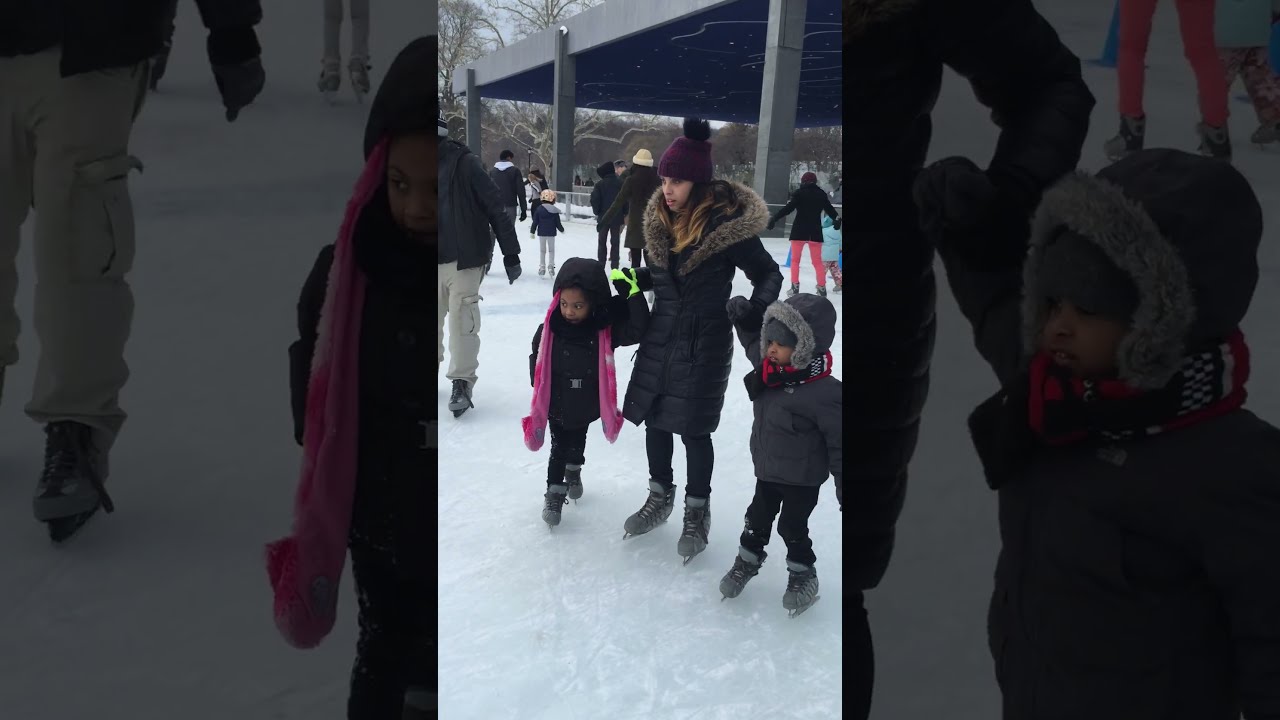In the photograph, a woman wearing a long puffer black jacket with a fur hood and a brown toque stands prominently in the foreground of an outdoor, snowy ice-skating rink. She is grasping the hands of two small children, both clad in black hooded coats with the hoods up and ice skates on their feet. The child on her right, a girl distinguished by her pink mittens, has her right arm extended downward while her left arm is raised, holding onto the woman’s right hand. She seems to be struggling to maintain her balance on the ice. On the woman’s left side, a boy, more stable in his stance, securely holds her left hand. The rink, bustling with other skaters, is surrounded by a scenic winter landscape of leafless trees, a hill, and an old-fashioned lamp post, all framed by a cloudy sky. A fence marks the boundary of the rink, with piles of snow visible at the base of the trees in the background.